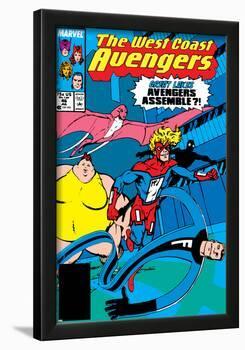The comic book cover features a black border framing "The West Coast Avengers" in bold yellow text with a red outline at the top. The modern Marvel logo is displayed in the upper left corner inside a blue box, which also contains four diverse characters—one masked figure and another potentially with a head-protective gear. A prominent pink pterodactyl-like creature with a face hovers at the top. Below this, a vibrant scene unfolds on a predominantly blue background. A massive woman in a tight yellow outfit stands imposing, while a golden-haired hero sporting a red and blue costume floats around her. An elastic, blue-outfitted superhero with a black "F" emblem, possibly from the Fantastic Four, stretches out across the bottom of the cover. Beside him, a shadowy figure reminiscent of Spider-Man adds to the dynamic lineup. A striking white speech bubble on the cover reads, "Great Lakes Avengers Assemble?!" in blue text, enhancing the intrigue. The overall electric composition vividly conveys the excitement and diversity of the Marvel universe.